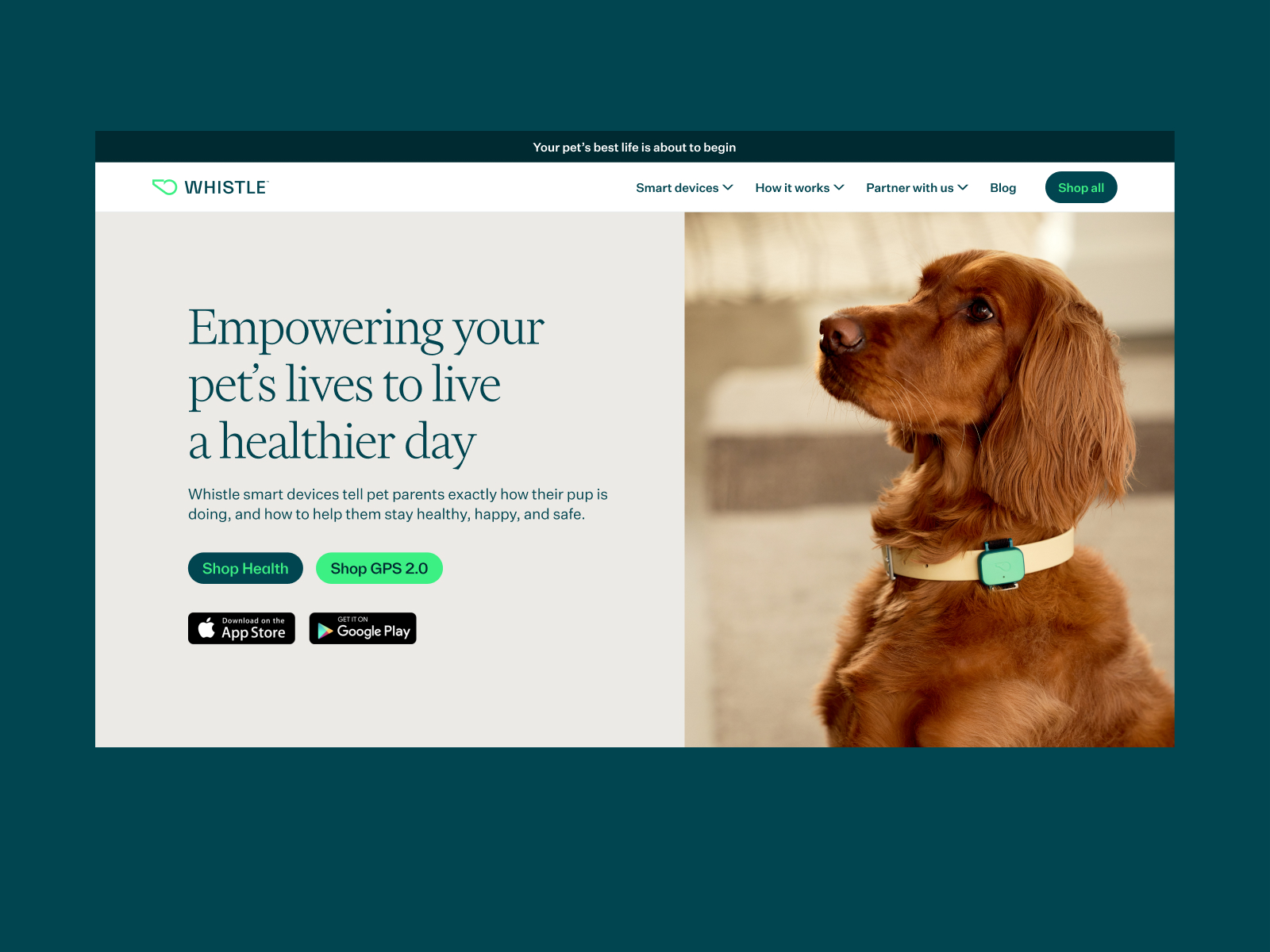The image features a sophisticated layout designed to promote pet wellness devices. The backdrop is a dark blue, transitioning into a black rectangle at the top center with bold white text stating, "Your pet's best life is about to begin." Below this, the header contains navigation elements on a white strip. On the left, there is an outline of a green whistle icon accompanied by the brand name 'Whistle' in black text. To the right, there are drop-down menu options labeled 'Smart Devices,' 'How It Works,' and 'Partner With Us,' followed by a 'Blog' link and a 'Shop All' button highlighted in blue text on a green background.

Further down, a section with a gray background holds a message on the left in black text: "Empowering your pet's life to have a healthier day. Smart Whistle devices tell pet parents exactly how their pup is doing and how to help them stay healthy, happy, and safe." Below the message are two buttons—'Shop Health' in blue text on a green background and 'Shop GPS 2.0' in green text on a blue background. The section also features the Apple App Store and Google Play Store logos, indicating app availability.

On the right side, there is an image of a golden retriever attentively gazing to the left. The dog is adorned with a white collar and a Whistle GPS tracking device, set against a modern kitchen background with white and tan shelving. This scene exudes a cozy, contemporary atmosphere, reinforcing the theme of pet health and safety in a home environment.